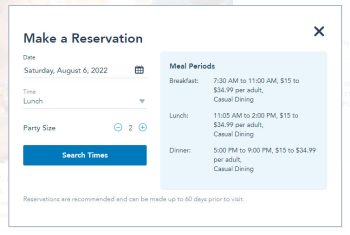This image is a screenshot taken from a website interface that allows users to reserve a table, though the specific website name is not identifiable. The design features a font reminiscent of OpenTable, but there's no direct mention of it. In the upper left corner, the interface prominently displays the text "Make a Reservation." Beneath this header, there are input fields designated for selecting the date, time, and party size. A blue rectangular 'Search Times' button is situated nearby for users to initiate their reservation search.

On the right side of the screen, a pale blue section titled "Meal Periods" in black font lists the different dining times available: Breakfast, Lunch, and Dinner. For each meal period, specific times and a cost per adult of $34.99 are indicated.

At the bottom of the screenshot, a very fine, pale gray font includes a note stating that reservations are recommended and can be made up to 60 days prior to the intended visit.